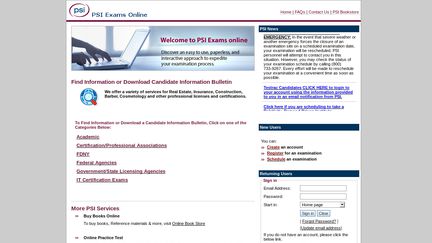The image depicts a blurry and grainy screenshot of a website named "PSI Exams Online," which is designed to facilitate online examinations. The website features a predominantly white background with black text, while some links appear in red and blue. The design and aesthetic of the website suggest that it may be relatively old. In the top right corner, there are red links for different sections, including "Questions and Answers" and "Contact Us." The top left corner of the site displays a small banner that reads "Welcome to PSI Exams Online" and includes an image of someone typing on an open laptop. Overall, the image quality is poor, making the details of the website difficult to discern.